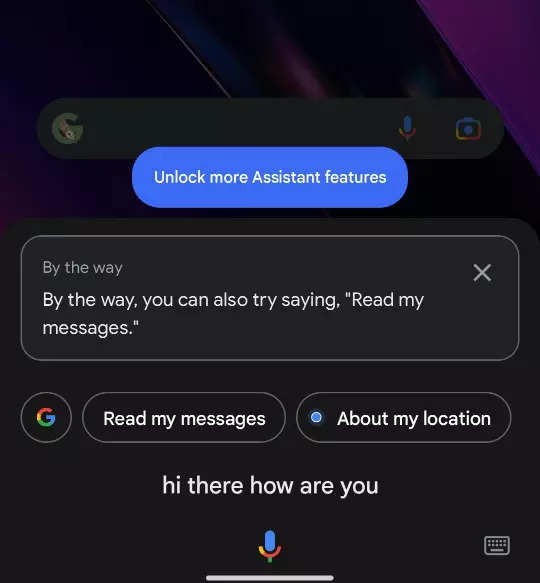The image depicts a user interface from a digital assistant app. At the top center, there's an oval-shaped blue box with the white text "Unlock more assistant features." Below this, a squared box appears on the top left with the heading "By the way," followed by the suggestion, "You can also try saying, read my messages."

In the middle section, there are three information bubbles. The first on the left is a circular icon with the Google logo, showcasing the colors red, yellow, green, and blue. The second bubble to the right contains the text "read my messages," and the third bubble says "about my location" with a small blue circle to its left.

Further down, the text "Hi there, how are you?" is displayed above a microphone icon situated at the bottom center. This microphone icon features the same blue, red, yellow, and green colors as the Google logo. Additionally, there's a gray keyboard icon positioned at the bottom right corner of the image.

For the background at the top half, there's a search bar. On the far left of the search bar, there is a green Google logo, while on the far right, there is a microphone icon and a camera icon, both featuring the blue, green, yellow, and red colors.